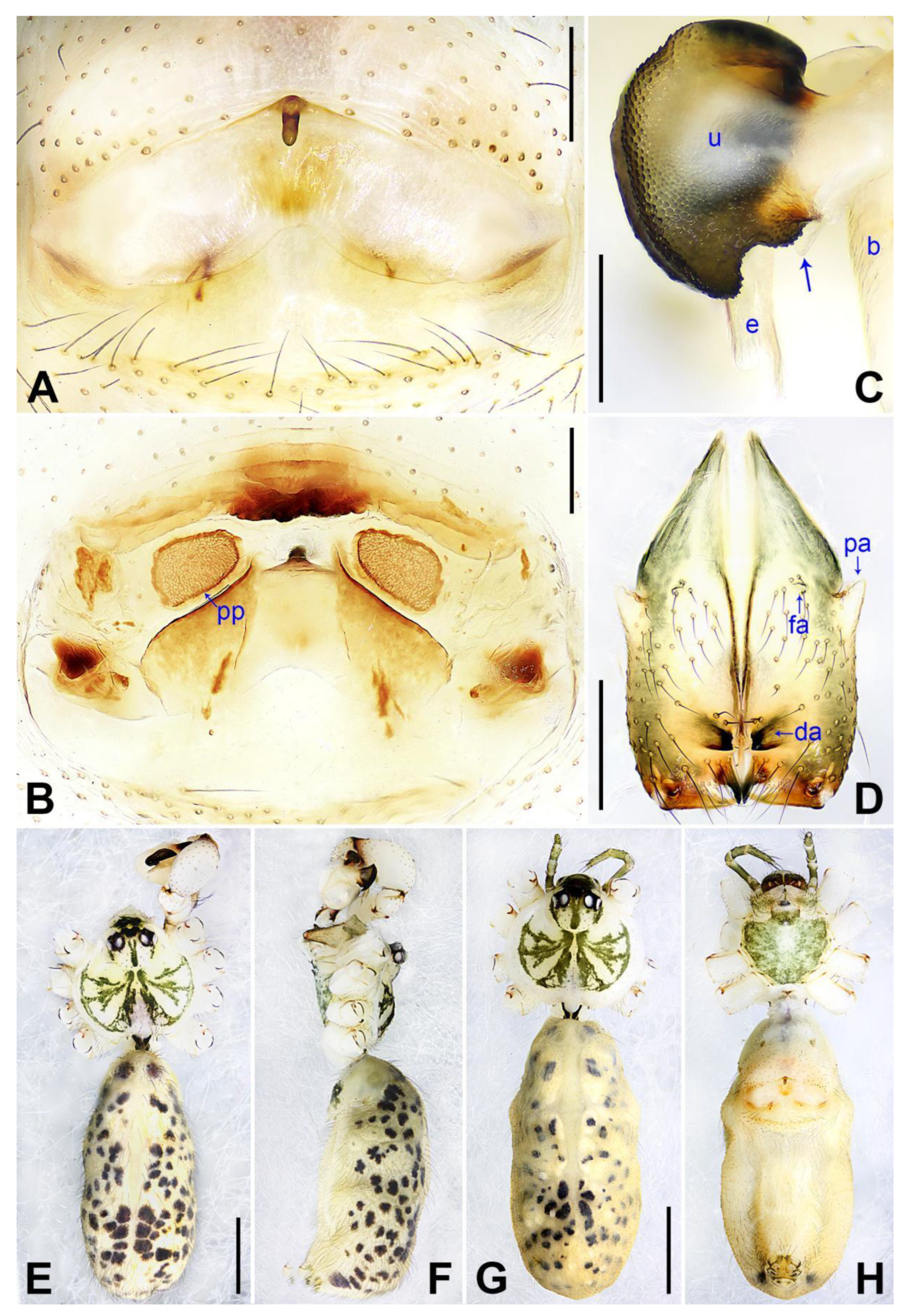The image is a detailed scientific diagram depicting the metamorphosis of an insect, possibly showing its transition into a cocoon. The layout consists of eight sections, labeled A through H, with four horizontal squares on the top row (A, B, C, D) and four vertical squares on the bottom row (E, F, G, H). The insect in the photographs, which is pale in color with green and black spots, has meticulously detailed visuals showcasing different parts and angles. The bottom row of images highlight the insect's head, body, and antennae, seemingly illustrating various stages of its emergence from a large sack, similar to a butterfly chrysalis. The remaining images appear to be detailed drawings of the same insect, though they are harder to identify specifically. One of these drawings, labeled C, features additional internal labels (U, E, and B) and displays a dark shape connected to a tan body part. The diagram also includes numerous unlabeled arrows and other figures like P, A, F, A, D, A, and P, P, adding to its complexity and potential use for educational purposes in a class presentation.